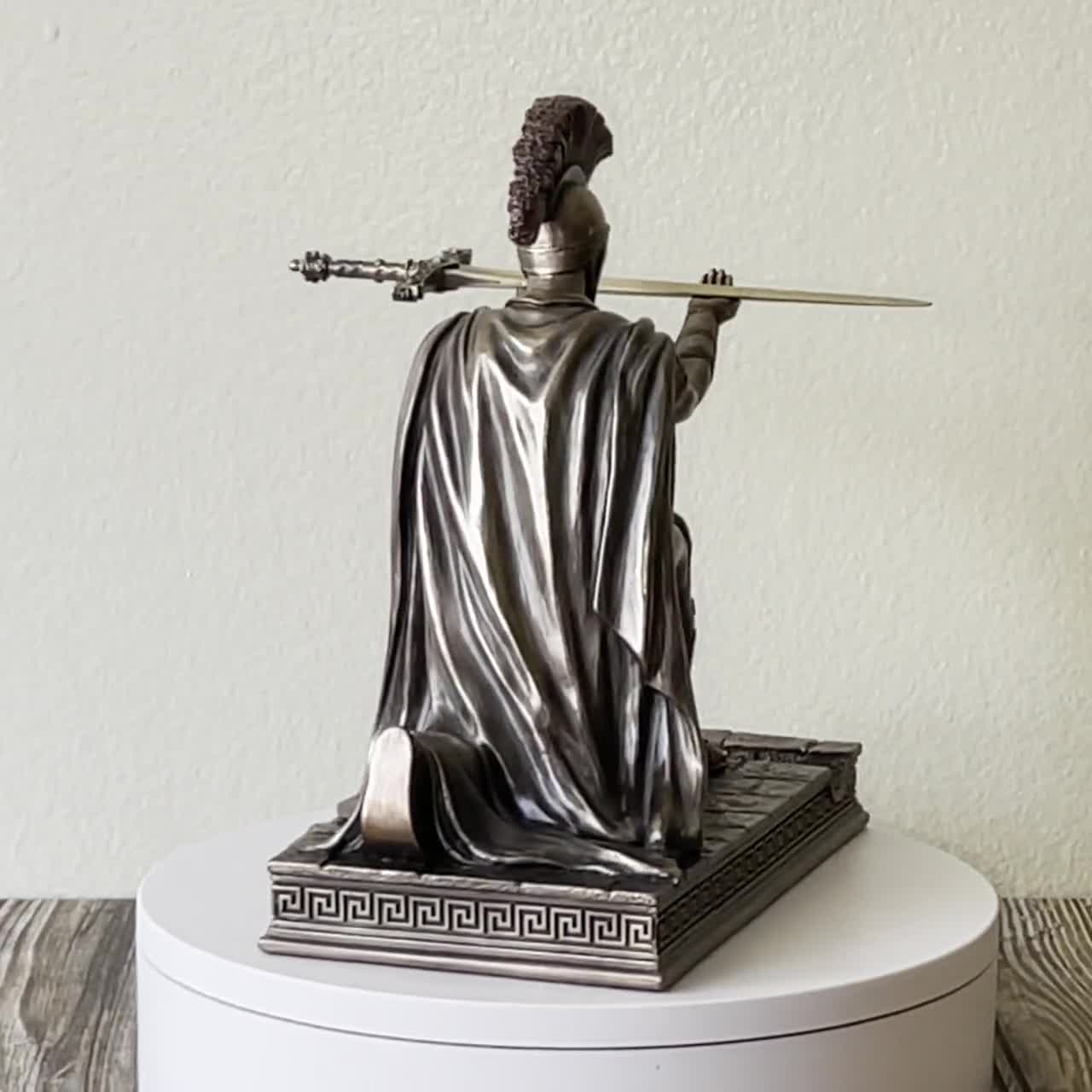The image depicts the back of a unique black statue of a Roman soldier, featuring intricate metalwork. The soldier, clad in a traditional Roman helmet adorned with a row of feathers from front to back, is kneeling on one knee on a pedestal. He is draped in a long flowing cape that cascades down his back. His outstretched hands hold a light sword, with a hilt that appears to be studded with jewels and a cross guard that is similarly adorned. The pedestal, crafted from inlaid stone, showcases a decorative design along its edge. The statue is positioned on a white circular base atop a wooden parquet floor, against a backdrop of pristine white walls. The detailed craftsmanship and the juxtaposition of materials create a striking visual effect in the display.